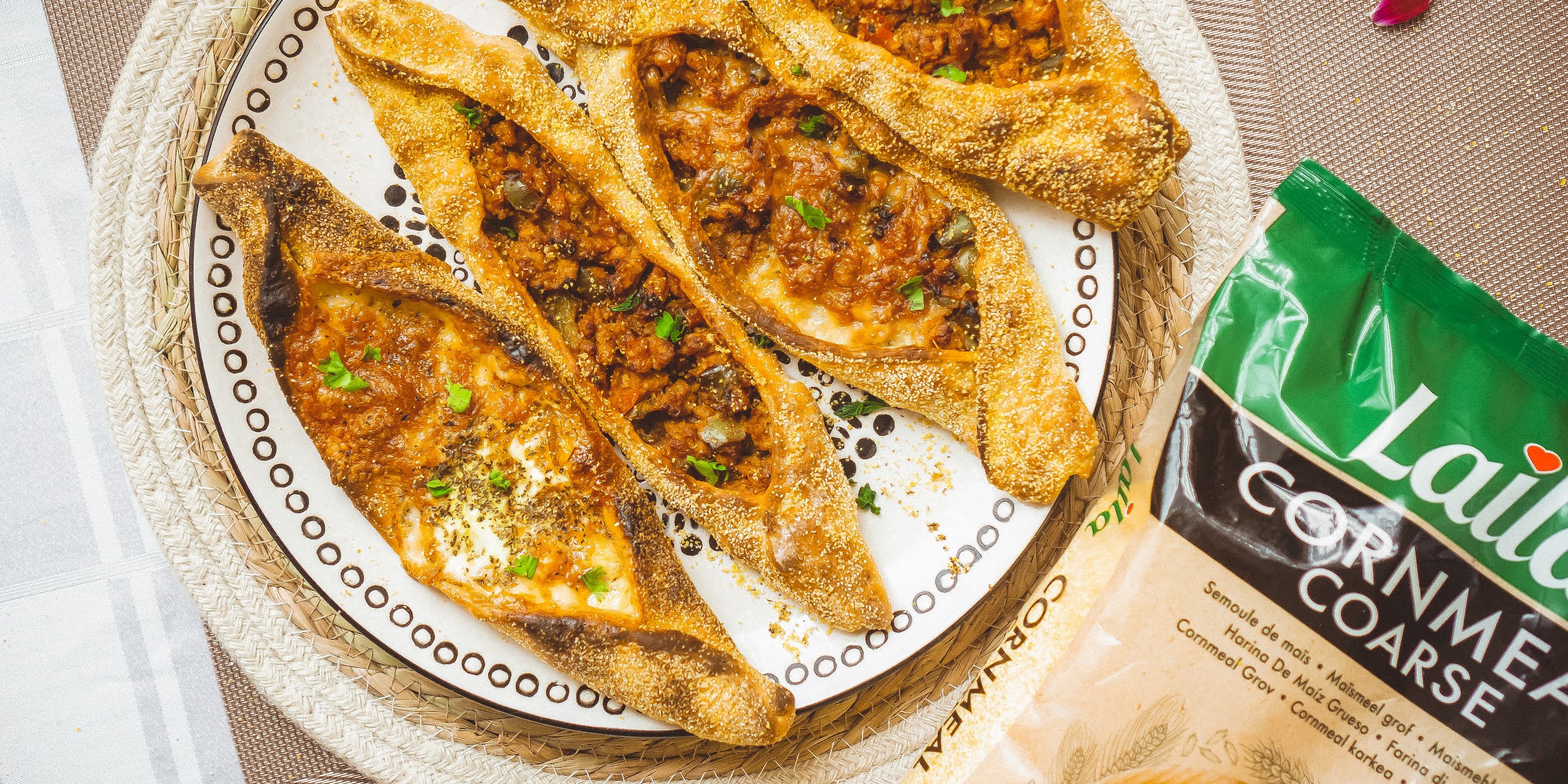In this vivid restaurant scene, a white ceramic plate is the focal point, featuring four boat-shaped pastries filled with a delicious mixture of cheese, meat, and vegetables. The pastries are neatly arranged, presenting a mix of inviting brown and yellow hues with green leaves garnish on top. The plate is adorned with little brown circles along the edge and rests on a light yellow wicker placemat. The entire setup sits over a white, thread-like woven surface. To the left of the plate lies a neatly folded white linen napkin, adding a touch of elegance. On the bottom right, partially intruding into the frame, is a green and brown package of coarse cornmeal. The packet, which has a bright green top with the word "Lail" and a red heart above the "i," further emphasizes the rustic yet vibrant atmosphere of the dining experience. The photograph, taken from above, captures the detailed textures and colors, making the dish look incredibly appetizing.